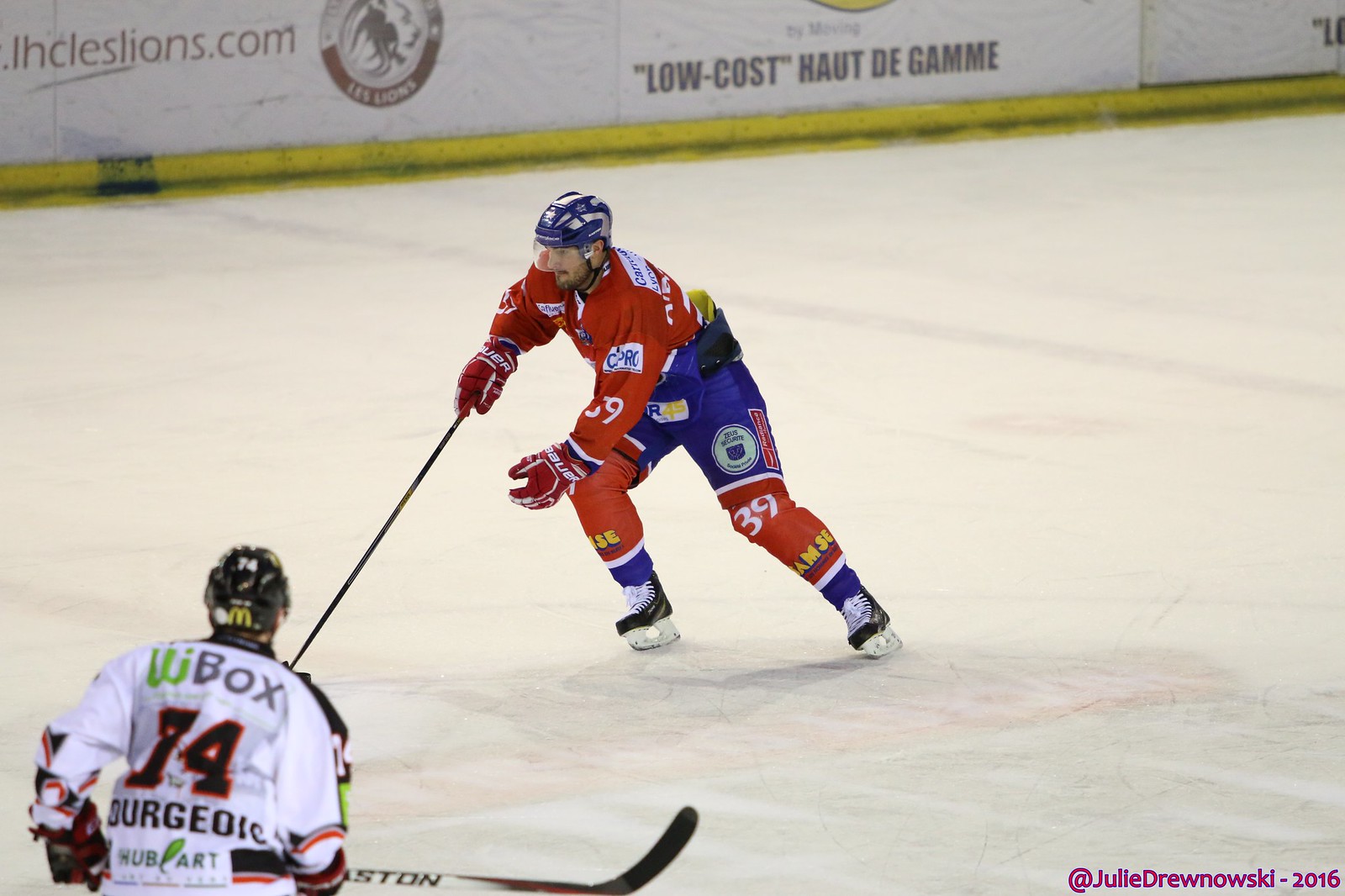This photograph captures an intense moment on an ice hockey rink, featuring two players in action. The rink's surface is a pristine white, with a boundary wall adorned with advertisements. The player in the foreground, numbered 39, is donned in a striking red jersey with blue accents, matching blue shorts, red gloves, and a blue helmet. His uniform is heavily padded, including red socks that extend up to his knee pads, and his skates are black. His opponent, with his back to the viewer, wears a white jersey numbered 14. The scene suggests a competitive event, possibly professional or a lower league, as the older players seem geared up meticulously. The bottom right corner of the image features a pink watermark that reads "@Julie Dronovski - 2016." Text in the background of the image reads "Low Cost Hot the Game."